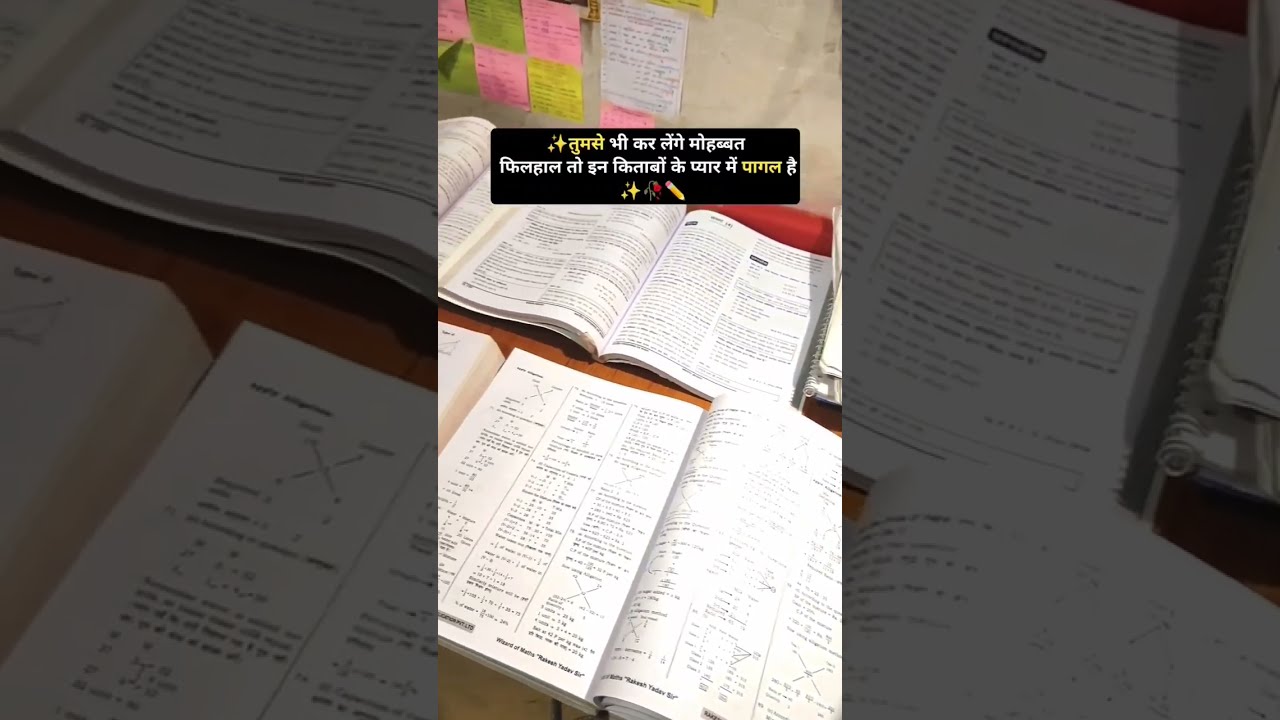This image shows an overhead view of a desk or table featuring two open textbooks, possibly three, which appear to be academic in nature, with one clearly being a math book, potentially focusing on trigonometry or geometry, evidenced by visible graphs and formulas. The table is set against a wall adorned with multiple colored sticky notes in white, pink, yellow, and green, suggesting a busy, organized study or classroom environment. At the top of the image, there is a prominent black horizontal rectangle containing text and symbols in a South Asian language, likely Hindi, and interspersed with star, rose, and pencil emojis. The main photo is oriented vertically, complemented by two smaller portrait images on either side, providing close-ups of the textbooks against a dark, opaque background, enhancing the overall composition into a landscape rectangle shape.